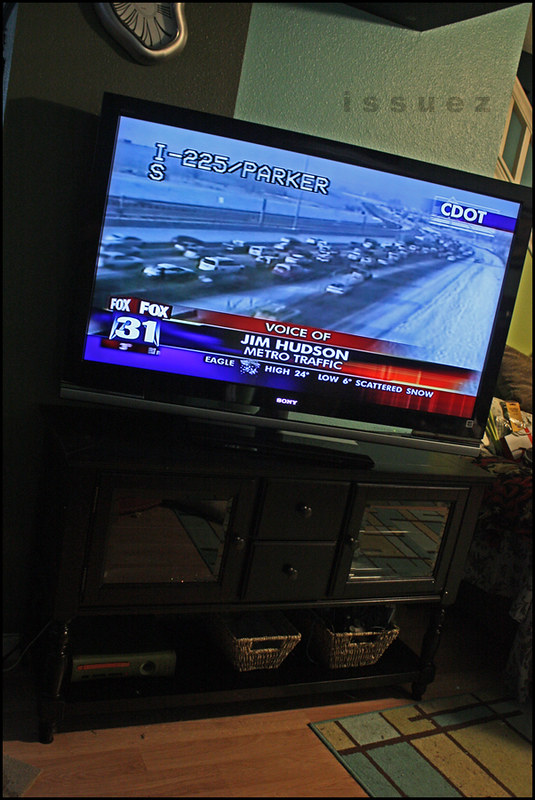The photograph captures a cozy interior setting of a home, framed by the focal point of a rectangular-shaped television screen prominently positioned on top of an organized TV stand. The stand itself features several shelves, accessorized with neatly placed items and a couple of small baskets at the bottom. The TV screen displays a live news broadcast from Fox 31, where the Voice of Jim Hudson reports on an intense traffic congestion, depicting a road densely packed with cars in gridlock. The bottom left corner of the screen is marked with Fox 31’s logo, rendered in striking red, white, and blue hues.

In the background, a partial glimpse of the home’s décor is visible. To the far right, the image hints at a staircase railing, subtly suggesting the layout of the home's interior architecture. In the top left corner, a portion of a clock—resembling the melting clocks reminiscent of Salvador Dalí’s surrealistic art—adds an intriguing and artistic accent to the scene. The combination of the detailed elements within the home and the informative broadcast on the television collectively encapsulates a moment balancing domestic tranquility and worldly awareness.